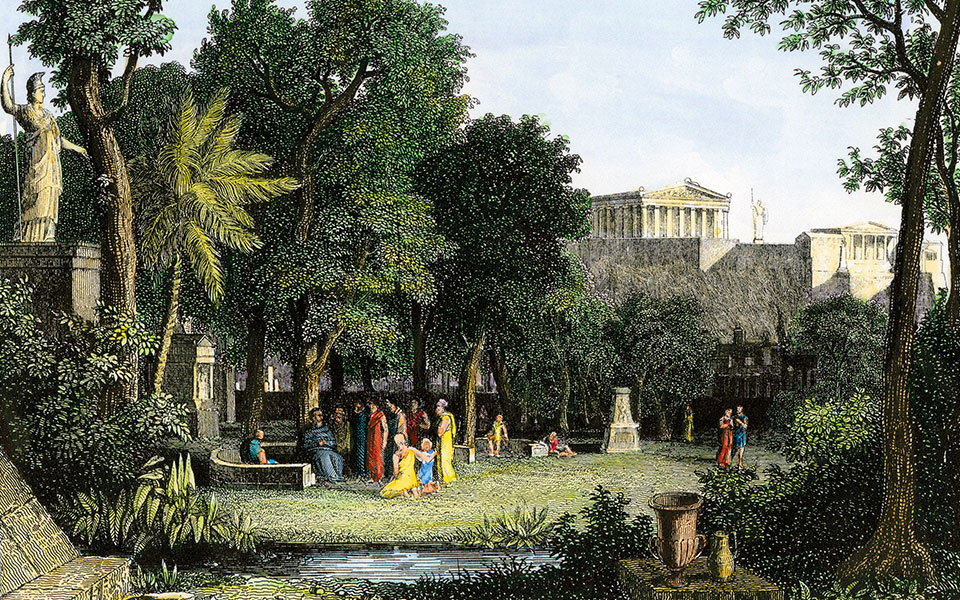The image portrays a detailed, drawn scenery set in ancient Greece, encapsulating a secluded area richly adorned with trees. In the center-left, a dark gray platform features a man standing confidently with a spear in one hand and the other hand outstretched, dressed in elaborate toga robes and a small helmet. This foreground is populated with a crowd, possibly students or followers, gathered around the central figure, perhaps a philosopher, eagerly listening to him. 

To the left and slightly above this gathering, statues reminiscent of ancient Greek artistry are prominent, signifying the historical context. In the background, stretching across the center to the far right, majestic Greek or Roman architectural structures, including Parthenon-type buildings, rise against the sky, with another statue nestled between these edifices.

The setting is lush with diverse trees, including a thick-trunked tree topped with abundant leaves and a slender palm tree. Additional robed figures are dispersed throughout the scene, some further in the back, possibly observing the gathering with curiosity or amusement. A small pond lies in the foreground, reflecting the serene, sunlit afternoon atmosphere, hinted by the shadows cast by the surrounding elements.